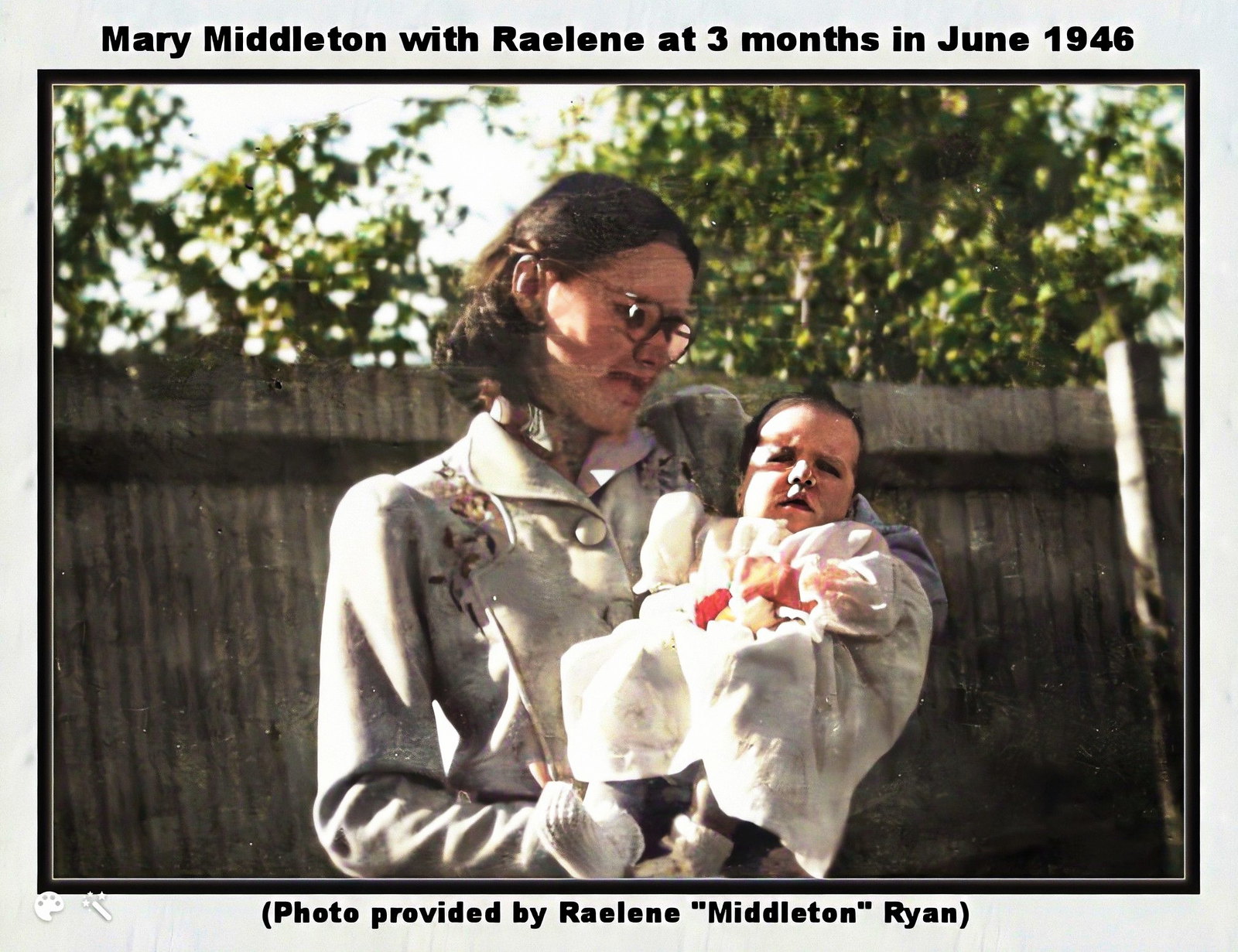In this vintage photograph captured in June 1946, Mary Middleton is seen lovingly holding her three-month-old baby, Raylene. The heartwarming moment is preserved with a caption in black text at the top of the image, reading "Mary Middleton with Raylene at three months in June 1946." A note at the bottom credits the photo's provision to Raylene Middleton Ryan. Mary is dressed in a grey coat, which contrasts gently with Raylene's warm, white baby clothes. They are standing in the sunny backyard of their family home in Piers, bordered by a charming wooden fence and framed by lush, green trees beyond. Mary, who is wearing glasses, gazes affectionately at Raylene with a broad, loving smile, making this a cherished family moment.